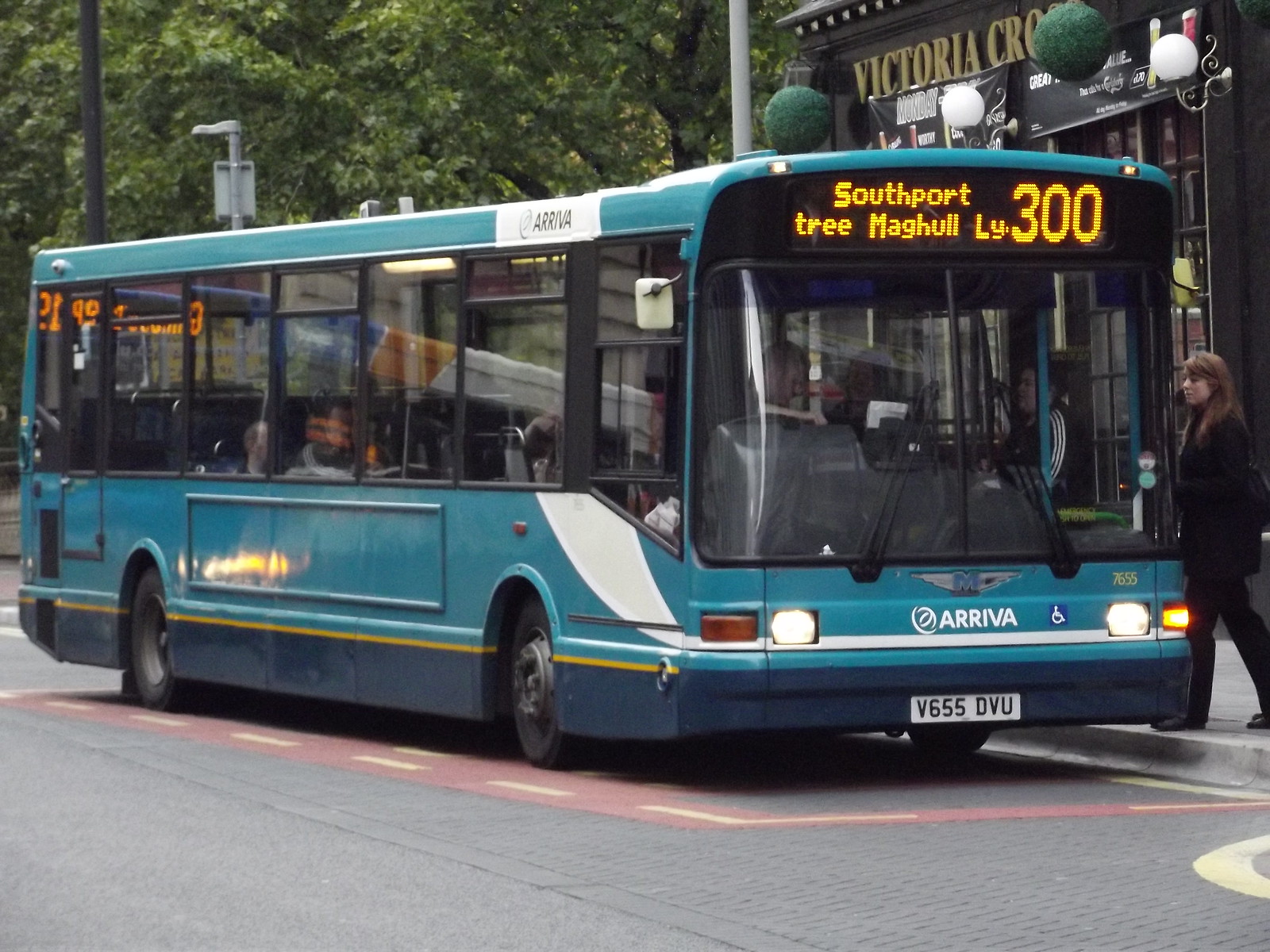This landscape-oriented color photograph captures a detailed urban scene centered around a teal blue public transit bus with white and yellow highlights, prominently featuring the name "Arriva" in white font on the front below the windows. The bus occupies almost the entire width of the image and is stationed in a designated parking area with distinctive red borders. Above the bus's headlights, a light-up sign reads "Southport Tree Magle LY300," accompanied by the number 7655 and a manufacturer's logo resembling an "M." A license plate, marked V655DVU, adheres to European standards.

To the right edge of the photo, a white woman with long brown hair, dressed entirely in black, is seen boarding the bus. She looks to be in her late twenties or early thirties. The scene is set in a bustling downtown shopping area, with storefronts featuring notable gold signages and white globe lanterns. One of the visible signs reads "Victoria Crow," though partially obscured by a green globe. In the background, lush trees provide a contrast to the urban environment. The photograph showcases a style of Photographic Representationalism Realism, capturing the vivid details and dynamics of everyday city life.